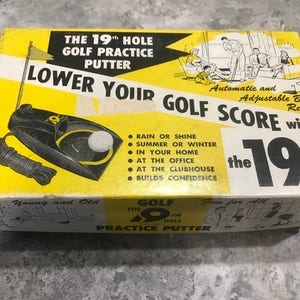This image displays an old and worn yellow and white box, slightly dented, containing a 19th Hole Golf Practice Putter kit. The box features a black flag graphic at the top, with white text reading "19th Hole Golf Practice Putter." A white ribbon diagonally spans the box, proclaiming "Lower your golf score with." Beneath this, central black text details various settings for use: "Rain or shine, summer or winter, in your home, at the office, at the clubhouse, builds confidence," each preceded by bullet points. The lower left corner of the box displays an image of the electric putting device, consisting of a black base with an AC plug and a circle at the end holding a golf ball, adjacent to a raised flag. On the upper right corner, a cartoon illustration shows a man putting indoors with family members observing – a woman in a chair, another person on a couch, and a child eagerly sitting on the floor. This portable device is advertised for versatile use, highlighting its ability to be plugged in and used virtually anywhere.